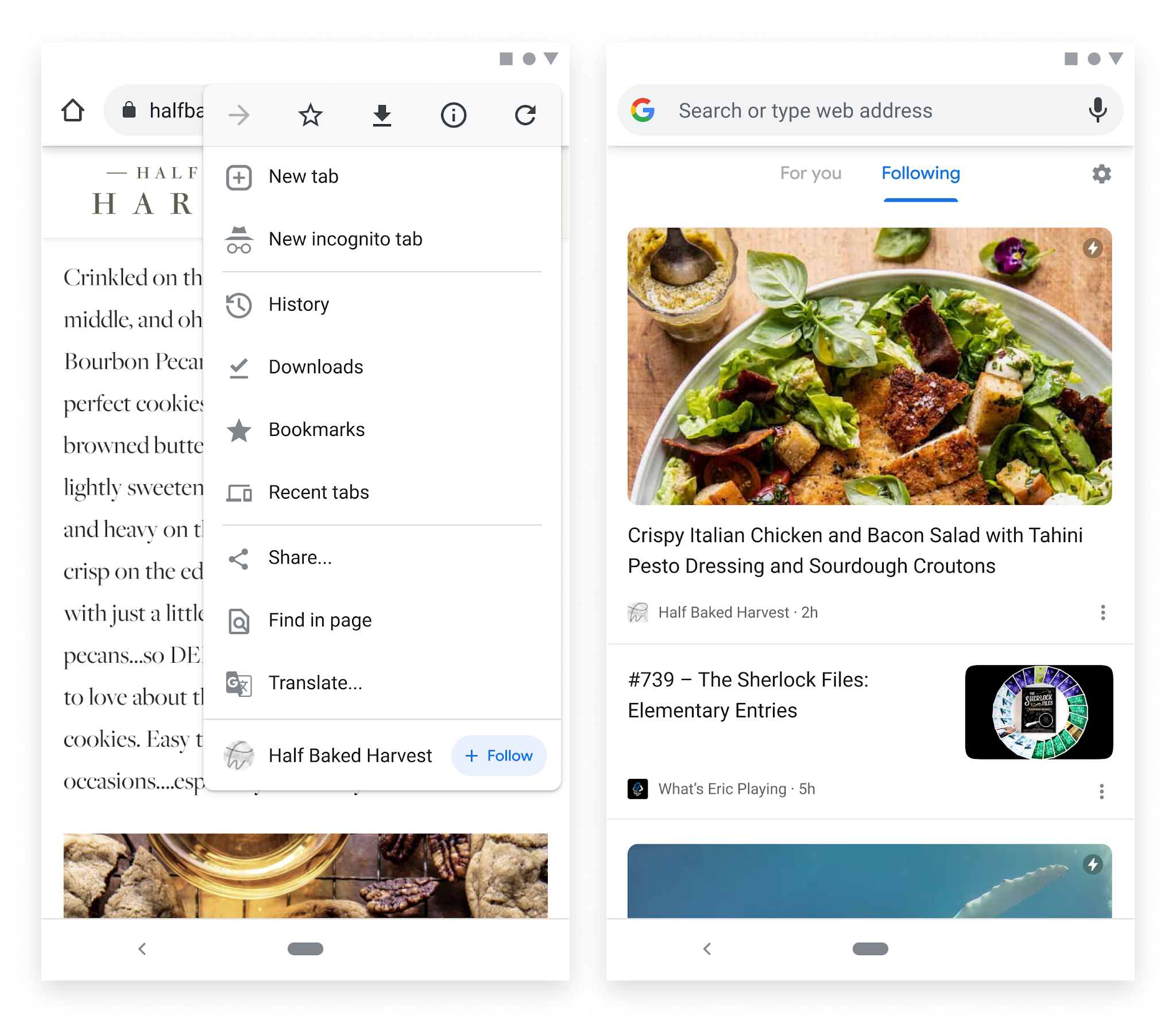On a mobile phone screen, two website pages are displayed side-by-side against a white background. 

Starting on the right-hand side, there is a prominent gray oval box featuring the Google "G" logo on the left side. This box includes the text field "Search or type web address." Below this, two tabs are visible: one labeled "For You" in gray, and another labeled "Following" highlighted in blue, with the username "Angelina Blue" also in blue. Adjacent to these tabs, there is a small gray gear icon, symbolizing settings.

Below the tabs, there is an appetizing image of a salad presented on a wooden table. The dish comprises chicken, croutons, and bacon, captioned "Crispy and Tired Chicken and Bacon Salad with Tahini Pesto Dressed in Sourdough Croutons." Below the image, "Have Baked at Harvest 2H" is fine-printed in gray. Beneath this, there is a horizontal gray line followed by a black text string resembling a web address or link, partially obscured: "pound key to 739-the-sherlock-files-autometry-entries."

The content continues with a highlighted question in black text: "What's Eric Playing 5H?"

On the left side of the screen, there is a white pop-up box. This box partially obstructs the underlying content and features several control icons: a right-pointing arrow, a star, a downward arrow, a circle with a black dot resembling an eye, and a refresh icon represented by an arrow creating a circle. Below the icons, the options are listed: "New Tab," "New Incognito Tab," followed by a horizontal line. The list continues with "History," "Downloads," "Bookmarks," "Recent Tabs," another horizontal line, "Share," "Find Page," "Translate," and an indication of additional options with "dot, dot, dot."

Beneath the pop-up box, the page shows content related to "Have Baked at Harvest" with the number "5H" in blue, signifying either the time or an identifier.